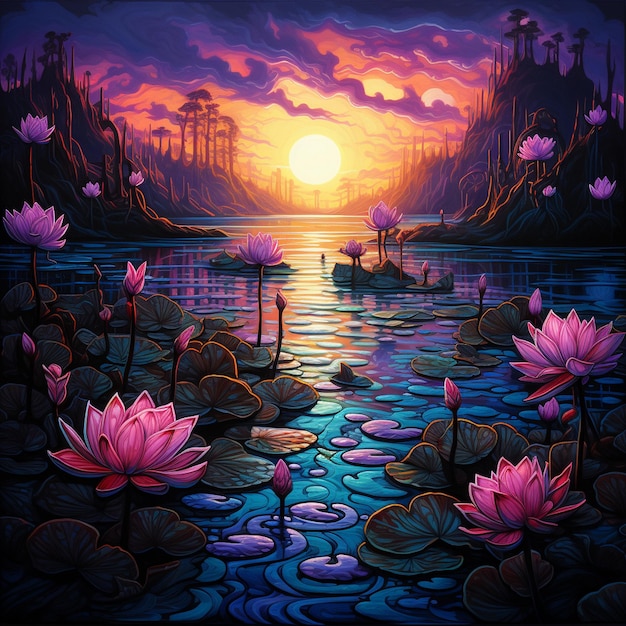This fantasy-style painting vividly captures a surreal night scene around a mystical pond. Central to the image, a large yellow sun is either rising or setting, casting vivid shades of orange and yellow across the sky. The sky is adorned with wispy, wavy clouds in hues of purple, dark blue, and orange, creating an eerie yet enchanting atmosphere. The surface of the pond is a mesmerizing mix of blue and purple swirls, dotted with lotus flowers and water lilies in shades of pink and purple. Dark green, shiny leaves float on the water's surface. The pond is bordered by round, dark banks that rise up gently on either side, leading to distant, artistically-rendered mountainous ranges covered in long, squiggly trees. These barren-looking trees add to the otherworldly ambiance of the scene, making the entire composition both eye-catching and immersive.